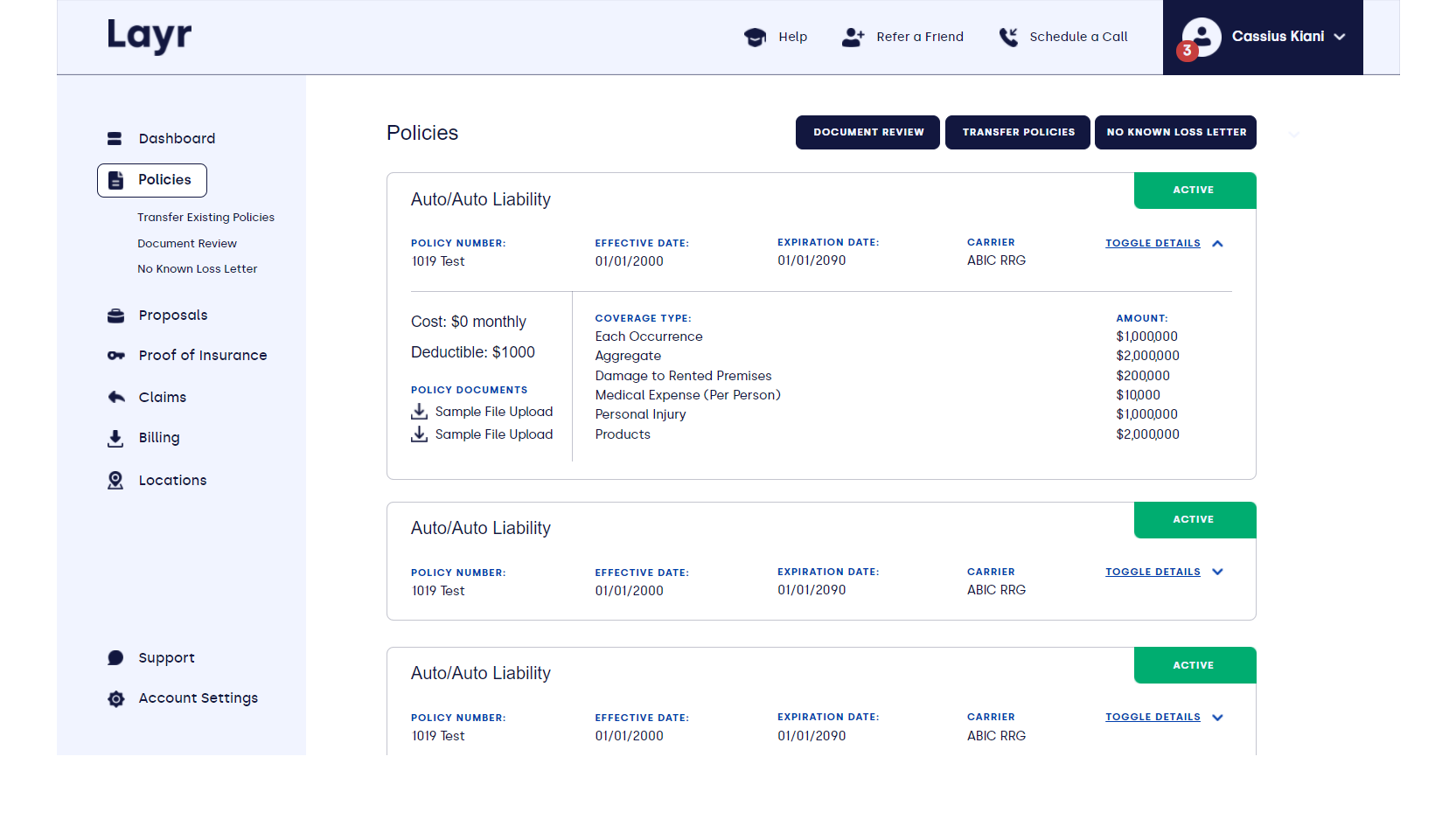The screenshot displays a white interface with a prominent purple overlay. It includes various sections: "Help," "Refer to a Friend," "Schedule a Call," and a profile icon. Below these options, the user's first and last name are visible.

The policy information section is detailed as follows:
- Policies: Auto / Auto Liability
- Status: Active (indicated by a green rectangle)
- Policy Number: [Some number]
- Effective Date: 01/01/2000 (slightly blurred)
- Expiration Date: 01/01/2090 (slightly blurred)
- Carrier: [Some letters]
- Toggle Details: Available
- Cost: $0 Monthly
- Deductible: $1,000

The coverage type section lists various coverage options and their corresponding amounts.

To the right, another section reiterates:
- Auto / Auto Liability status (Active, displayed in a green rectangle)
- Policy Number: [A number]
- Effective Date: (repeated information)

Overall, the interface provides a comprehensive overview of the user's auto liability policy, including coverage details, costs, and contact options.